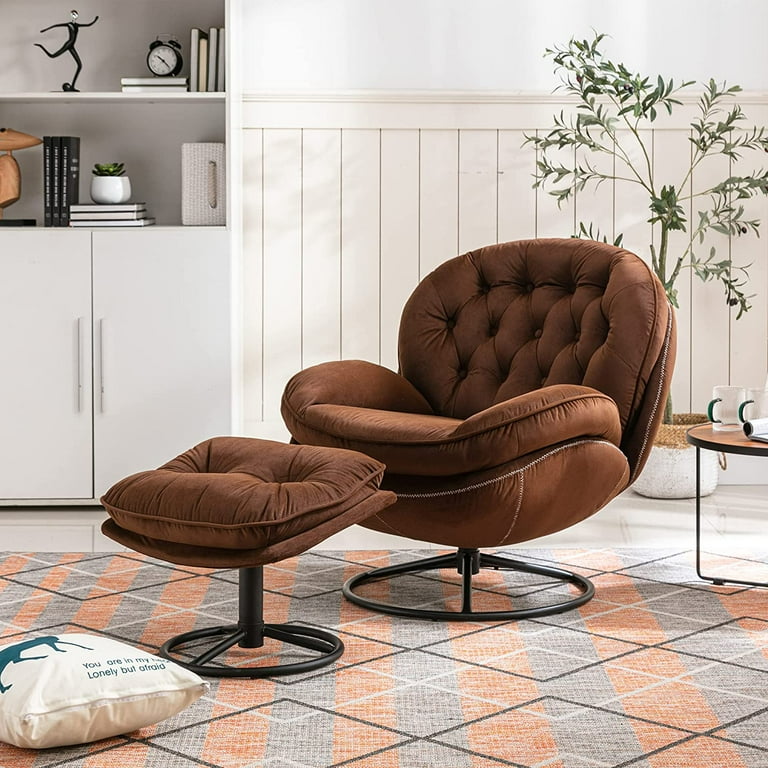This close-up indoor image showcases a plush, bowl-shaped brown chair accompanied by a matching footstool, both featuring a round base connected to a thick rod allowing for swivel movement. The footstool sports a thick pillow, complementing the chair’s apparent softness, likely covered in a velvety material. In front of the footstool, a white pillow with a bluish-green silhouette and writing adds a touch of personalization, though the text's exact words are partially unreadable—mentioning "You are in my [blank], Lonely but afraid." The seating arrangement rests on a geometric rug characterized by orange, gray, and interwoven white and black lines creating a striped pattern.

Behind the chair, a large green plant with a white base and burlap wrapping sits, adding a natural element to the scene. Adjacent is a small wooden nightstand with thin steel supports, positioned near a storage cabinet with large white doors. Atop the cabinet, a stack of books and a small planter with a plant enhance the homey atmosphere. Another set of upright books with white writing adds to the literary feel, while an additional burlap-colored storage bin with a handle is visible to the right.

The overall background is predominantly white, with white paneling and bookshelves holding various books and statues, completing the room’s decor.